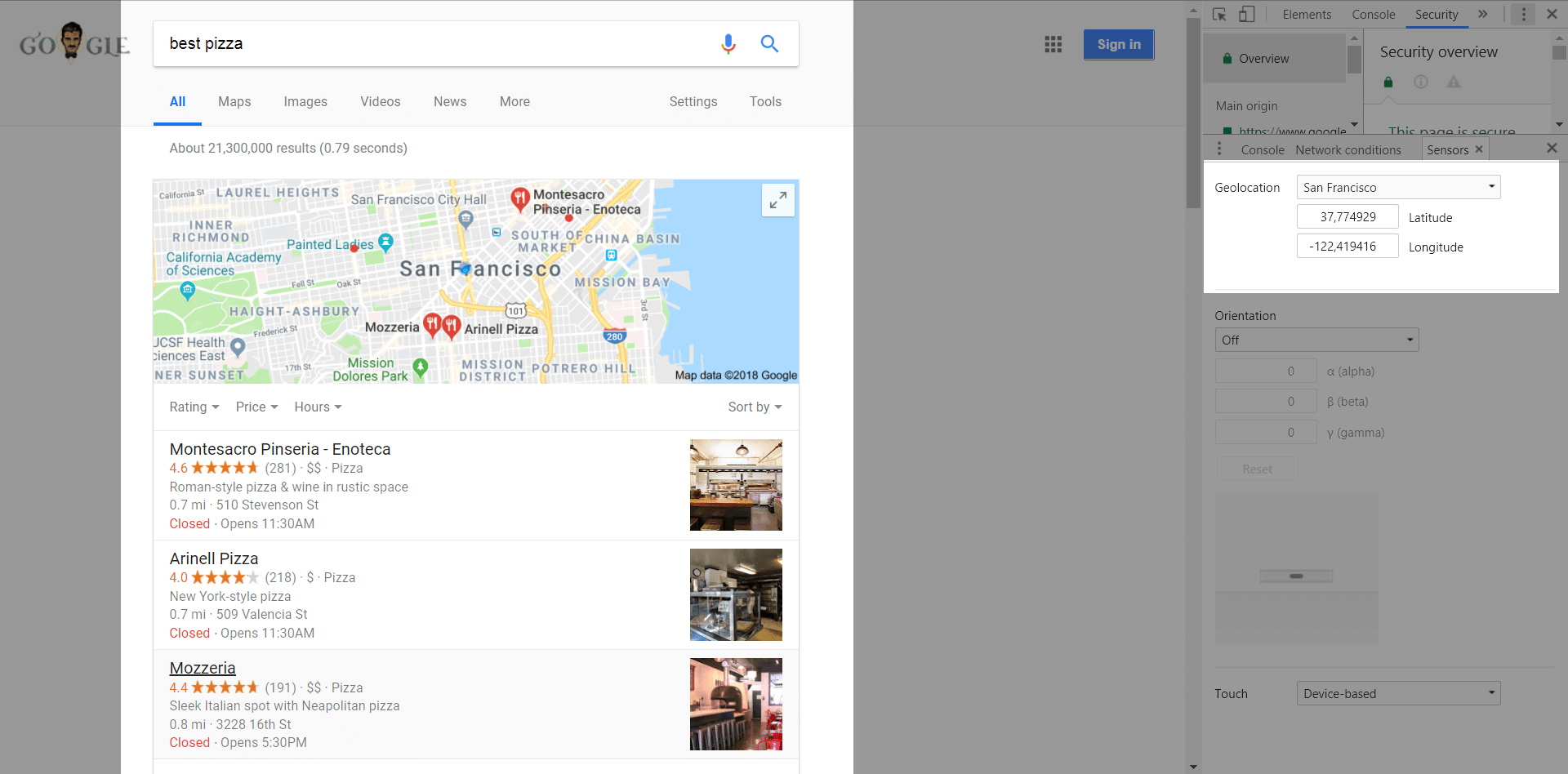This image is a screenshot of Google Maps with a search for "Best Pizza" focused on San Francisco. The map displays an overhead view of the city streets with minimal detail, marked with several red pins indicating various pizza restaurants. The central part of the map clearly labels "San Francisco," and the ocean is visible to the right.

Three pizzerias are listed below the map:

1. **Montesacro Pizzeria**:
   - Rating: 4.6 stars
   - Description: Roman-style pizza and wine in a rustic space
   - Currently Closed: Opens at 11:30 AM
   - A small image of the restaurant is provided to the right of the description.
   
2. **Arenal Pizza**:
   - Rating: 4 stars
   - Directions and operating hours are available but not fully visible in the screenshot.

3. **Mozzeria**:
   - Rating: 4.4 stars

All the highlighted pizza restaurants are marked with red pins on the map, showcasing their locations throughout San Francisco.